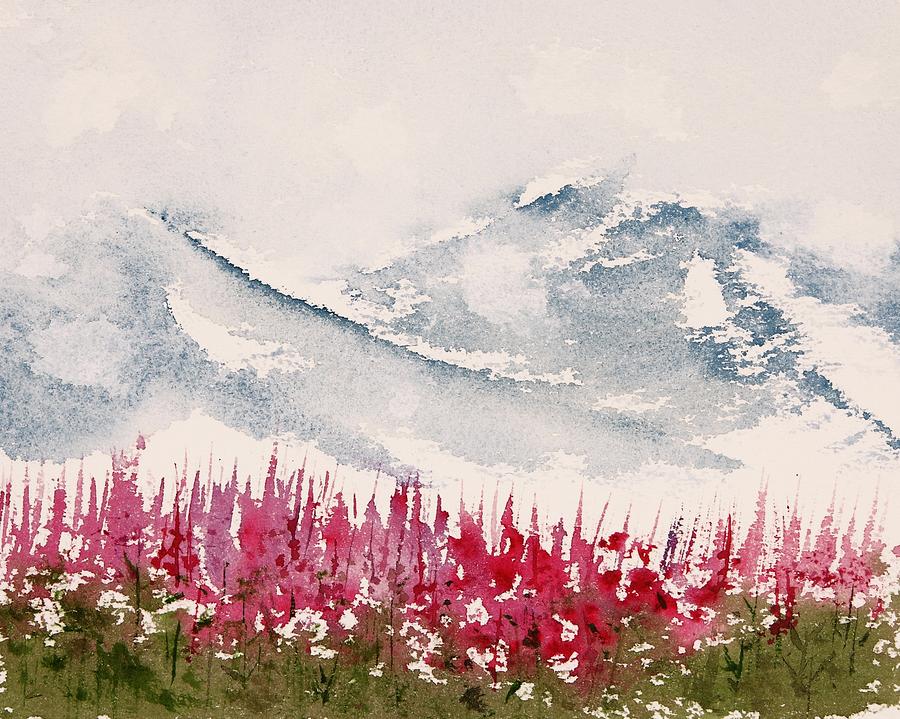This detailed sketch depicts a vibrant winter scene where towering, snow-capped mountains loom in the distant background. The mountains, illustrated using pastel crayons or chalk, exhibit extensive shading that suggests the presence of dark, forested areas amidst the snowy peaks. These majestic mountains are contrasted by the foreground adorned with tall, wildflowers swaying slightly as if caught in a gentle breeze. The flowers are depicted in a spectrum of pinks and reds, with some hints of lavender pink, standing on long stems with green leaves, rooted in a lush, grassy field. The sky, rendered in shades of gray and light blue, adds a serene yet cloudy ambiance, enhancing the painting's abstract quality. Despite the wintry scene suggested by the snow-covered mountains, the vivid colors of the flowers and field create a striking, unusual juxtaposition of seasons within a single, cohesive artwork.